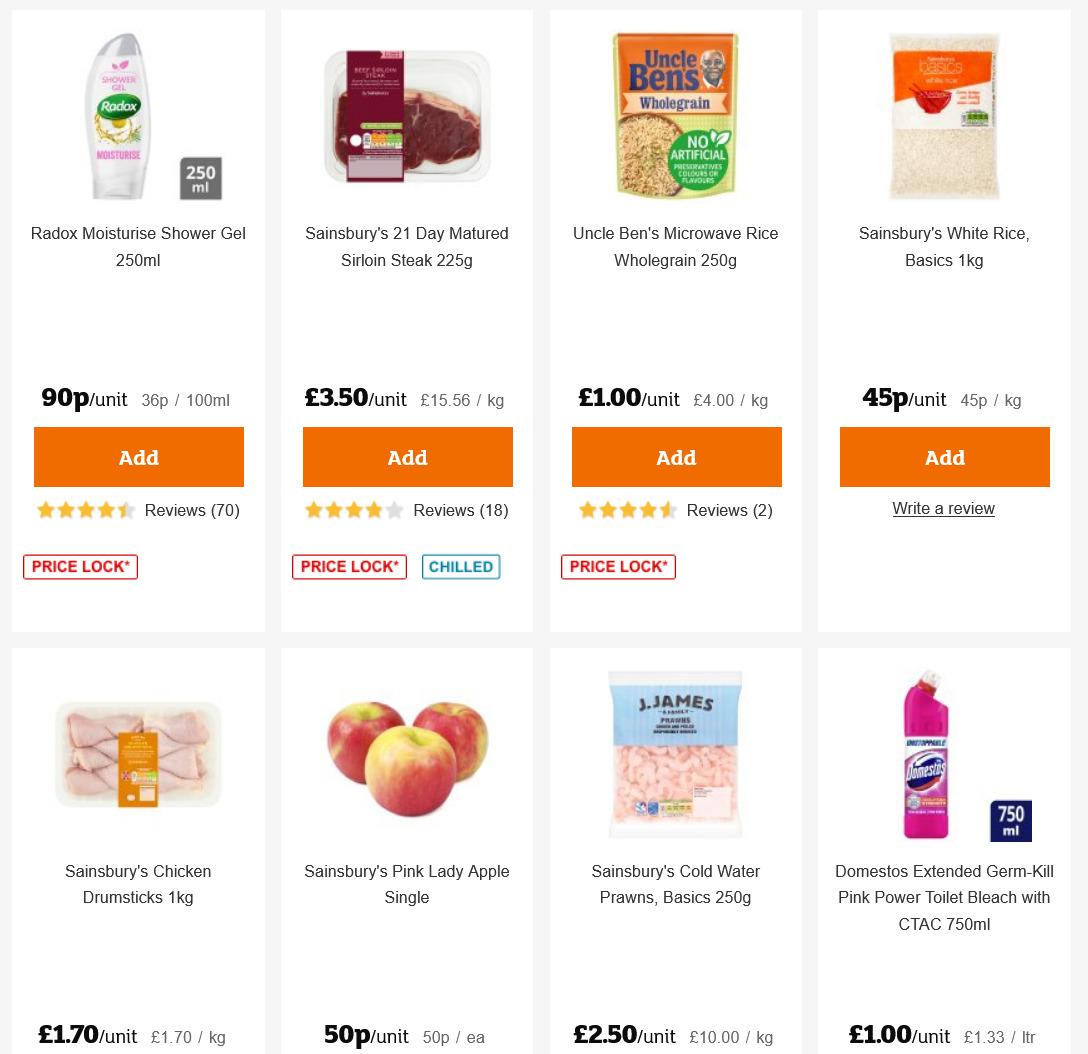### Detailed Description of Shopping Website Screenshot

The screenshot displays a shopping website page featuring a grid layout with two rows, each containing four items. The layout is slightly clipped, showing the top row completely and only the prices of the items in the bottom row. Here's a detailed breakdown of each item's presentation:

#### Top Row:

1. **Radex Moisture Shower Gel**
   - Volume: 250 ml
   - Price: £0.90 per unit, £0.36 per 100 ml
   - Features: A white and pink bottle
   - Rating: 4.5 stars from 70 reviews
   - Labels: Orange "Add" button, Red "Price Lock" tag

2. **Sandsberry 21 Day Matured Sirloin Steak**
   - Weight: 225g
   - Price: £3.50 per unit, £15.56 per kg
   - Features: Chilled, shown in burgundy and white packaging with a teal icon
   - Rating: 4 stars from 18 reviews
   - Labels: Orange "Add" button, Red "Price Lock" tag

3. **Uncle Ben's Microwave Rice Whole Grain**
   - Weight: 250g
   - Price: £1.00 per unit, £4.00 per kg
   - Features: Golden-orange packet
   - Rating: 2 reviews
   - Labels: Orange "Add" button, Red "Price Lock" tag

4. **Sandsberry White Rice Basics**
   - Weight: 1kg
   - Price: £0.45 per unit, £0.45 per kg
   - Labels: Orange "Add" button, "Write a Review" prompt

#### Bottom Row (partially visible):

5. **Sandsberry Chicken Drumsticks**
   - Weight: 1kg
   - Price: £1.70 per unit, £1.70 per kg
   - Features: Light pink drumsticks in white packaging

6. **Sandsberry Pink Lady Apples**
   - Price: £0.50 each

7. **Sandsberry Cold Water Prawns Basics**
   - Weight: 250g
   - Price: £2.50 per unit, £10.00 per kg

8. **Joe Manisto's Extended Germ Kill Pink Power Toilet Bleach with SeaTac**
   - Volume: 750 ml
   - Price: £1.00 per unit, £1.33 per liter
   - Features: Light pink packaging

Each item in the top row prominently features an orange "Add" button and a red "Price Lock" tag. The presented information includes product name, volume or weight, unit price, reviews, ratings, and special features. The bottom row items, though partially visible, include key details like price and some packaging descriptions. The overall interface appears to emphasize convenience and clarity in user interactions with easily accessible pricing, ratings, and purchasing options.